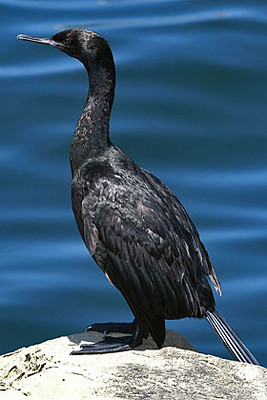This is a color photograph taken outside on a sunny day, featuring a close-up, profile view of an aquatic bird, likely a species of duck. The bird, predominantly black with a glossy sheen to its feathers, exhibits a narrow beak and a long tail. It stands on a large, light gray rock, its black webbed feet clearly visible against the stone surface. The bird's head and neck are duck-like, with its gaze directed to the left side of the image. Behind the bird is a calm, blue body of water, adding a serene background to the scene. The overall image is brightly lit, highlighting the clear details and textures of the bird and its surroundings. The photograph contains no additional animals, people, text, or vehicles, and the clarity suggests it was taken in natural daylight.